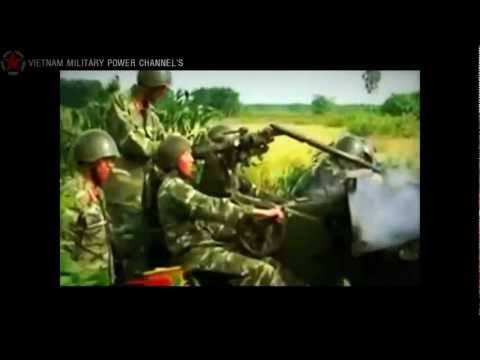The image features a photograph centered within a black background that forms a border around it, creating a rectangular frame. The photograph prominently displays three soldiers clad in green camouflage military uniforms and smooth, rounded green helmets. They appear to be operating a piece of army green machinery, possibly an anti-aircraft device, amidst a field that could be part of a wetland area. Visible in the background are green trees and an overcast sky, enhancing the scene's somewhat dreary ambiance. The soldiers and their equipment blend into the surroundings due to their camouflage, causing a slight blurring effect. At the top of the black border, in bold white letters, is the text "Vietnam Military Power Channel 8," accompanied by a red star to the left of the text. Despite the potential blur and chaotic nature of the scene, the photograph offers a vivid depiction of military action in a natural setting.